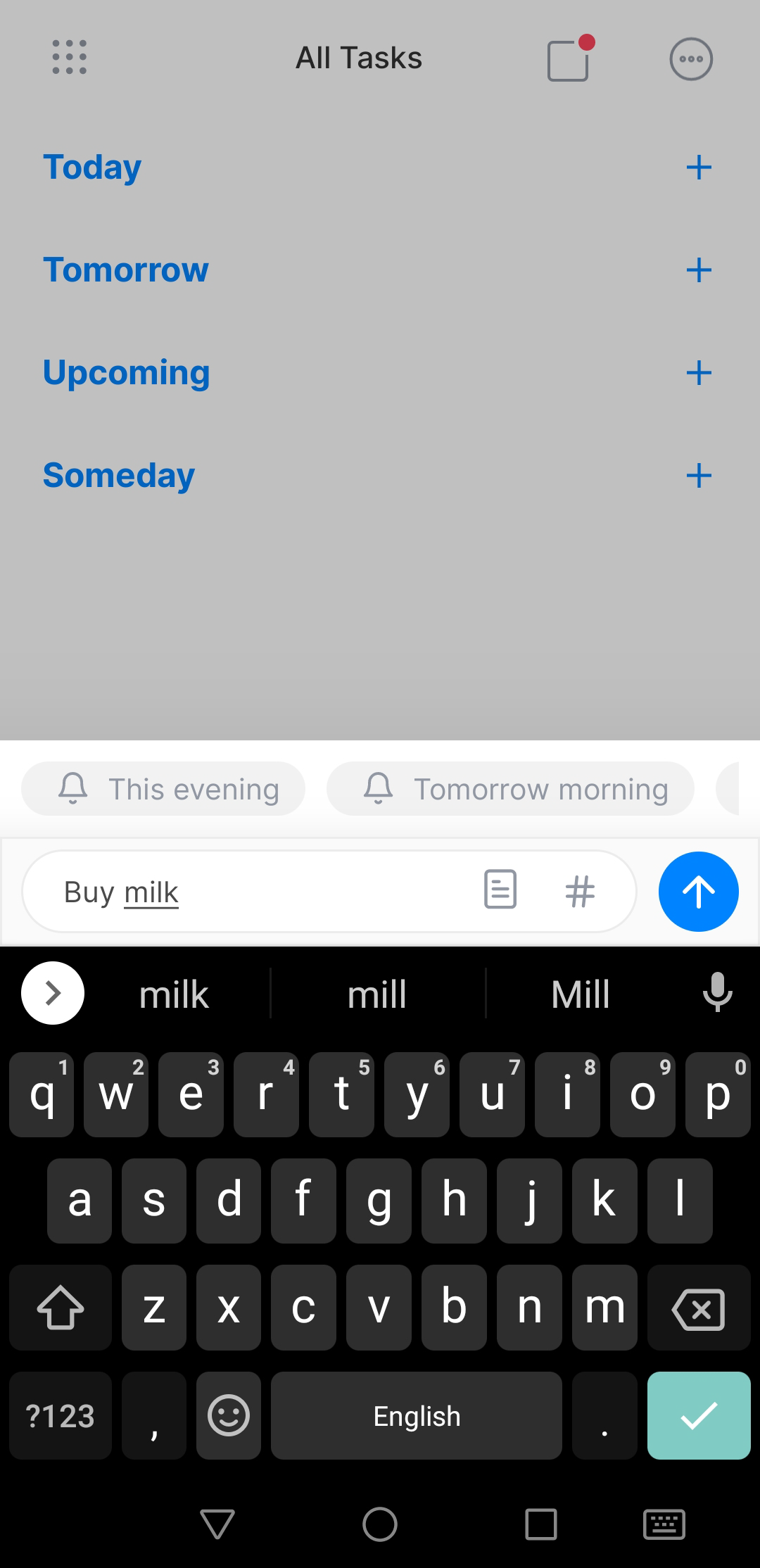This screenshot presents a detailed view of a task management application interface. At the top of the screen, a light taupe-gray square features a 3x3 arrangement of dots in the upper left corner. Centrally positioned in black text, the title "All Tasks" is prominently displayed, with both the 'A' in "All" and the 'T' in "Tasks" capitalized. 

Adjacent to this title on the right, there is a square followed by a line, and a small red circle appears at the top-right corner, likely indicating a notification or alert. Further to the right, there is another circle containing a horizontal alignment of three small dots.

Beneath this top section, there are four vertically stacked sections labeled "Today," "Tomorrow," "Upcoming," and "Someday," each in blue text with the first letter capitalized (T, T, U, S). Each of these sections has a respective plus sign located directly to the right.

Below these categories, the interface extends to display two tabbed sections labeled "This Evening" and "Tomorrow Morning," each accompanied by a bell icon, suggesting scheduled reminders. Underneath these tabs, there is a search bar containing the text "Buy milk," with "milk" being underlined.

On the far right, a blue circle with an upward-pointing arrow is present, indicating an action such as submission or navigation. Finally, the bottom section of the screenshot features a standard keyboard layout for text input, showing the letters in their usual arrangement.